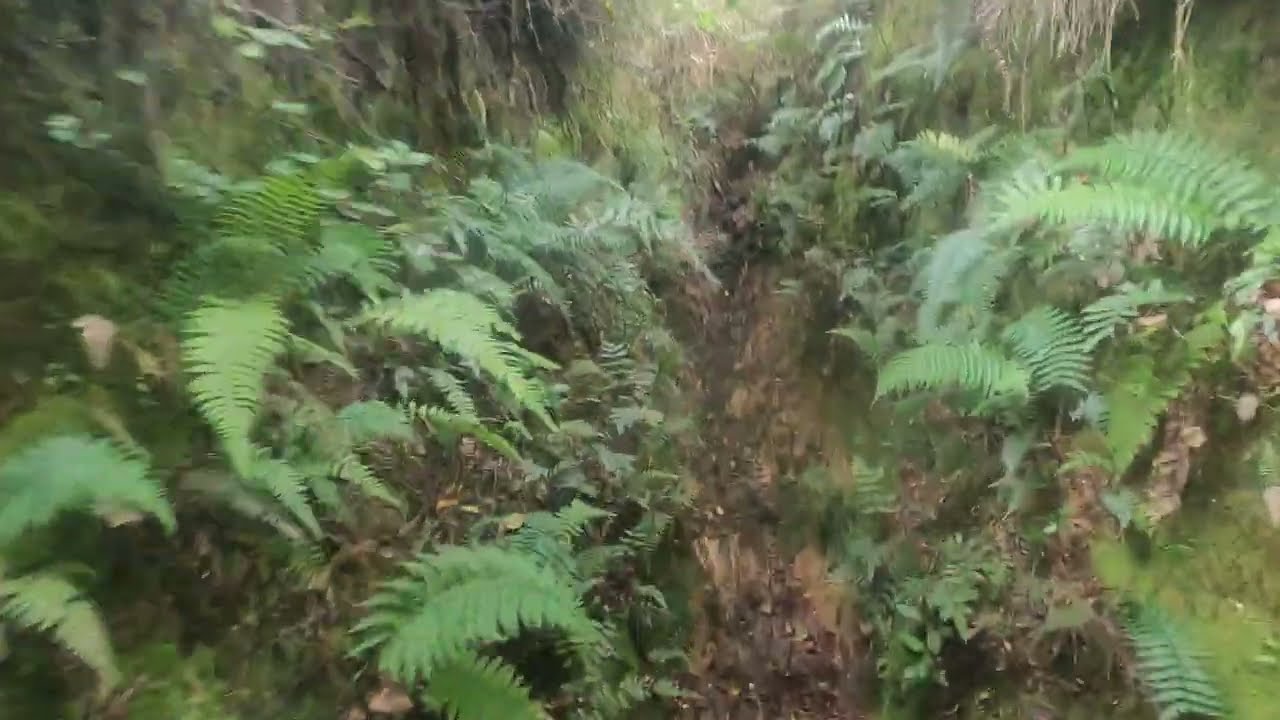This photograph appears to be an overgrown and heavily forested area, possibly in a rainforest or dense woodland environment. The scene is dominated by a mixture of bright green ferns and various shrubs that heavily obscure the narrow, barely-visible path cutting through the greenery. Surrounding the path, dense vegetation includes overlapping leaves, dark brown tree trunks, and decaying plant matter, such as wilted palm fronds and old yellow grasses. The ground seems muddy and littered with rocks, broken branches, and moss. The weather looks overcast, contributing to the image's muted colors of yellow, black, white, gray, and various shades of brown and green. The photograph is blurry, possibly due to movement or a lack of focus, and it captures no animals or people, lending an air of isolation and wilderness to the scene.